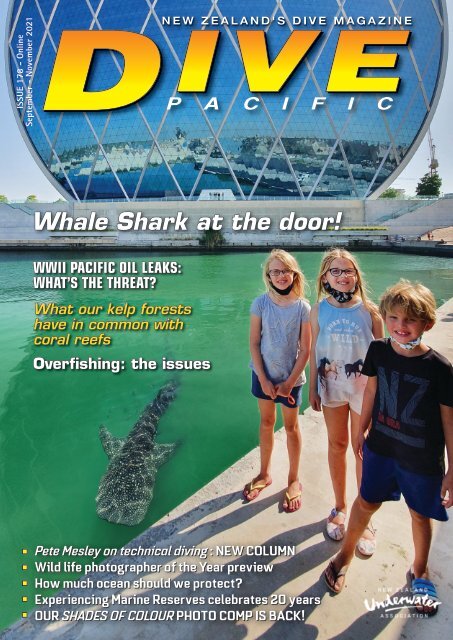This image is the cover of Dive Pacific, New England's dive magazine. At the top, there's bold yellow text that reads "DIVE" with smaller text above and below it stating "New England's Dive Magazine" and "Pacific." The cover features an intriguing photograph of three children standing on a concrete slab beside a pool of greenish water, staring at what appears to be a whale shark submerged in the water with only a portion of its body visible. The water is so clear that the tail end of the whale shark is discernible, while its head remains submerged. Additionally, there are several bullet points at the bottom detailing the contents of the magazine, such as "WWII Pacific Oil Leaks: What’s the Threat?" and "What Do Kelp Forests Have in Common with Coral Reefs?" along with discussions on overfishing. The issue is marked "Issue 178-online September to November 2021."